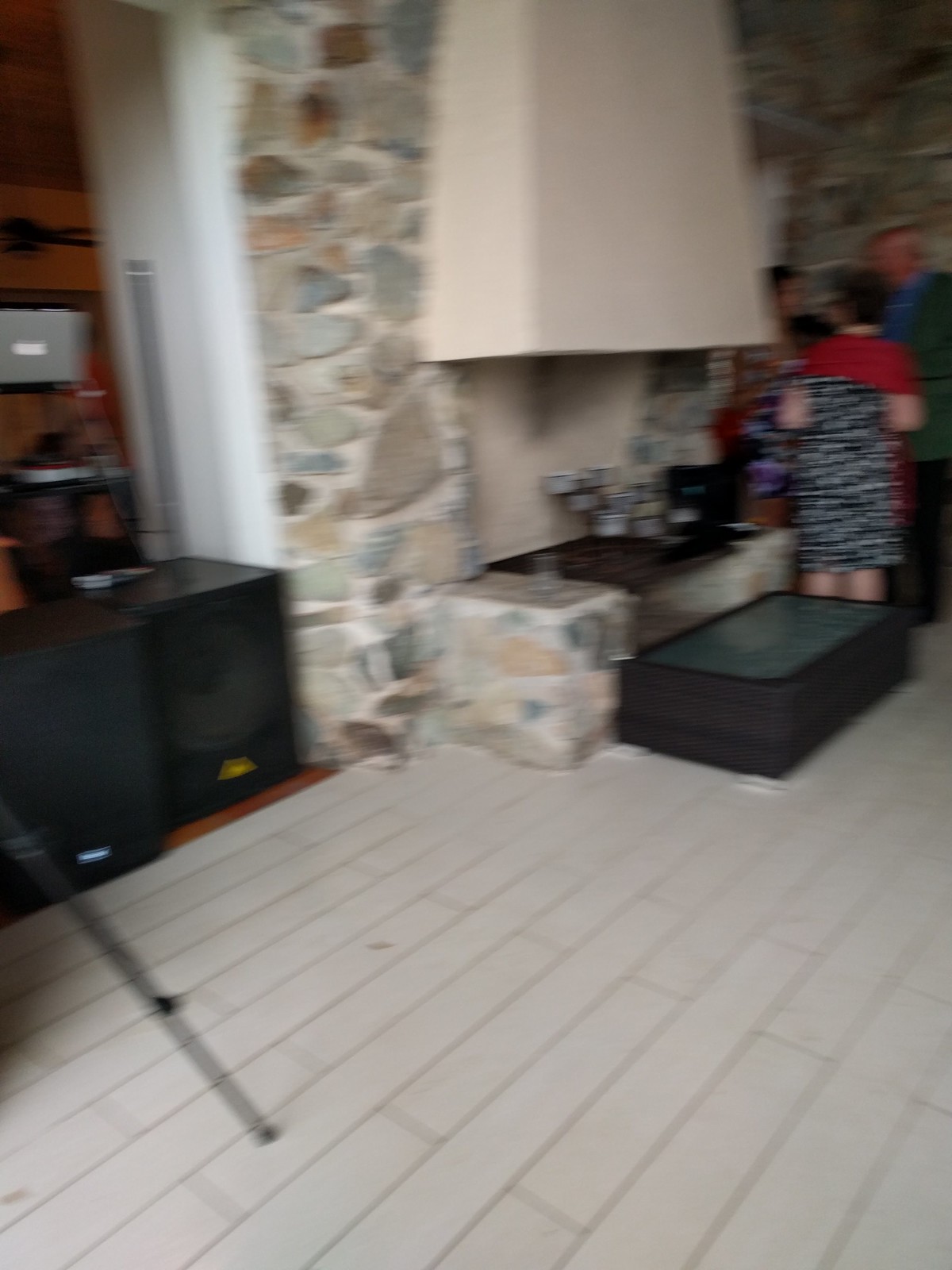A warm and cozy room features a wooden floor with white wood. At the top of the image, light smoke suggests the presence of a fireplace, subtly out of focus. Surrounding the fireplace are stone walls crafted from brown and gray stones with sections of white walls adding a contrast. On the far right, more stone structure is visible. In front of the fireplace, there is a raised platform with a wooden bench where people are gathered, engaging in conversation. They are dressed in black coats similar to ours, with striking red sashes draped over their shoulders. These individuals are positioned both to the left and right side of the bench. On the far left side of the image, a black counter is seen against more white walls. In the distant background, elements of wood can be observed, possibly indicating the presence of a monitor partially concealed within the décor.